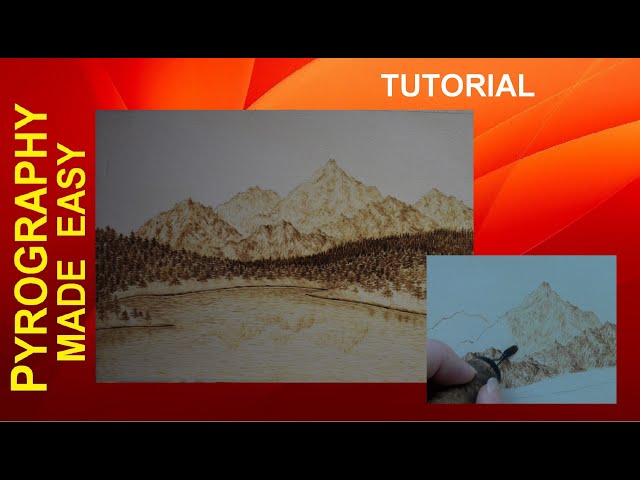The image is a screenshot from a PowerPoint presentation with an orange variegated background featuring numerous lines. Dominating the center is a detailed drawing depicting a serene nature scene with mountains, a dense forest, and a large body of water. The top right corner of the slide is labeled "Tutorial," while the left side displays the text "Pyrography Made Easy" at an angled orientation. In the bottom right corner, a hand holding a flat, dark brown pencil with a smooth, black pointed tip is actively drawing the mountains. The scene beautifully captures the essence of pyrography as an artistic technique.